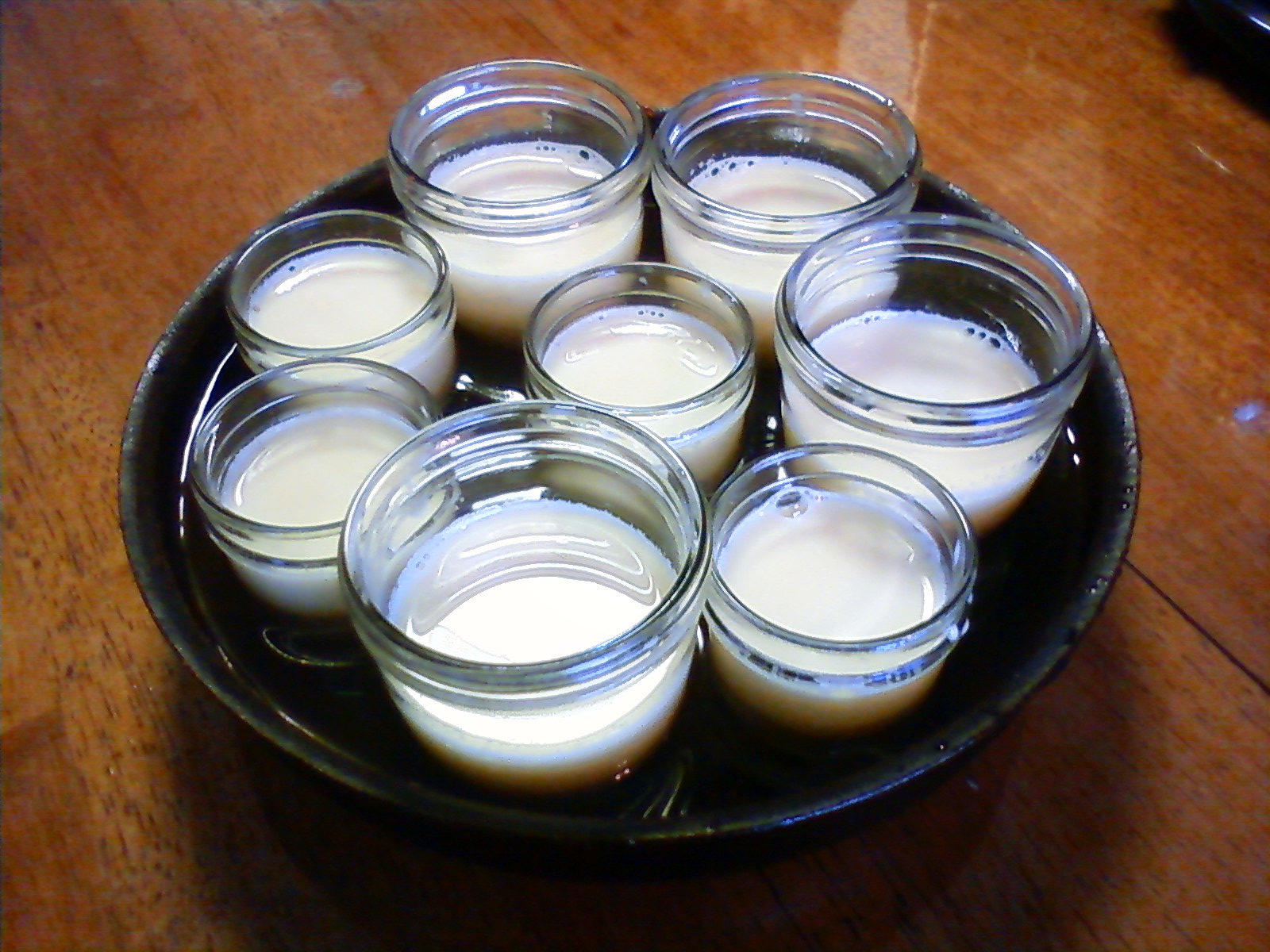In this indoor photograph, a rustic wooden table with a high-gloss finish serves as the backdrop. The table's medium-brown surface, with visible wood grains, reflects light in certain parts, enhancing its polished appearance. Centrally positioned on the table is a large, black tray, roughly one inch in depth, that holds several glass jars of varying sizes. Specifically, there are eight jars: one very large, three medium, and four smaller ones. Each jar is partially filled, ranging from halfway to three-quarters full, with a thick, opaque white liquid that resembles milk or cream. The jars, which have screw-top lids, are arranged neatly within the tray, some displaying minor bubbles within the creamy substance, suggesting a dense consistency.